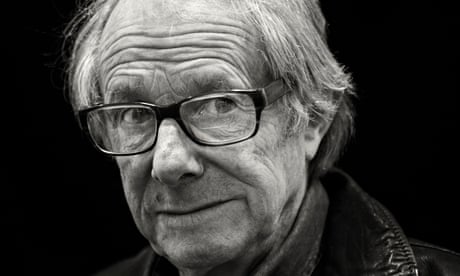This black-and-white photographic portrait features British director Ken Loach. The image is in landscape orientation, capturing him from the top of his forehead to just under his chin. Ken is depicted with shaggy salt-and-pepper hair, primarily bald on top, and wisps of longish gray hair around his ears and neck. He wears thick black-rimmed bifocals and a somewhat serious expression, looking slightly up and to the right, almost in a three-quarter profile.

Ken's face is marked by multiple wrinkles and furrows, particularly on his brow, and he has thin, long eyebrows. A noticeable mole sits above his lip. He is dressed in a layered outfit, featuring a shiny leather coat over what appears to be a denim shirt or jacket. The background is solid black, emphasizing the serious and posed nature of this portrait, which could easily be an author photo for a newspaper or a book jacket.